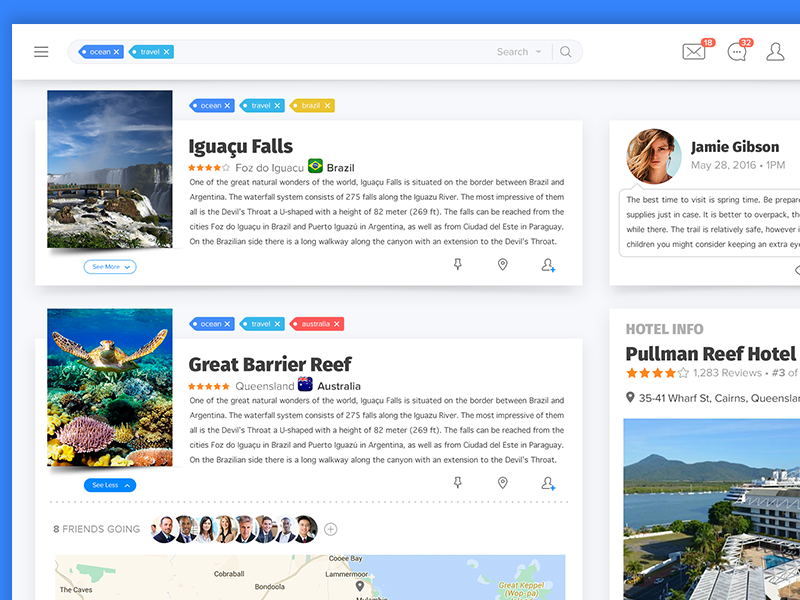Certainly! Here’s a clean and detailed caption for the described image:

---

The website features reviews of notable tourist attractions. On the far left, there are two vertically aligned photos. The first photo showcases a breathtaking outdoor scene with a sky and clouds backdrop, highlighting the majestic Iguazu Falls. This image is tagged with "ocean," "travel," and "Brazil." Prominently displayed beneath the photo is the text "Iguazu Falls," accompanied by a four-star rating. Additional details include "Foz do Iguaçu" with the Brazilian flag icon, indicating its location in Brazil. A brief description states: "One of the great natural wonders of the world, Iguazu Falls is situated on the border between Brazil and Argentina. The waterfall system consists of 275 falls along the Iguazu River. The most impressive of them all is the Devil's Throat, a U-shaped section with a height of 82 meters (269 feet). The falls can be reached from the cities Foz do Iguaçu in Brazil, Puerto Iguazu in Argentina, and Ciudad del Este in Paraguay. On the Brazilian side, there is a long walkway along the canyon, with an extension to the Devil's Throat."

Beneath this visual splendor, an underwater photograph captures a serene turtle swimming close to the ocean floor. This image is tagged with "ocean," "travel," and "Australia." The accompanying text "Great Barrier Reef" is highlighted in large font, coupled with a five-star rating, "Queensland," the Australian flag, and the description "Australia." Notably, the same review text used for the Iguazu Falls is repeated for the Great Barrier Reef, indicating a potential oversight.

On the right side of the page, there is an image of a woman named Jamie Gibson. Below her photo, there is information about the Pullman Reef Hotel, offering accommodations related to the reviewed locations.

---

This caption provides a comprehensive and organized breakdown of the image for clarity and context.